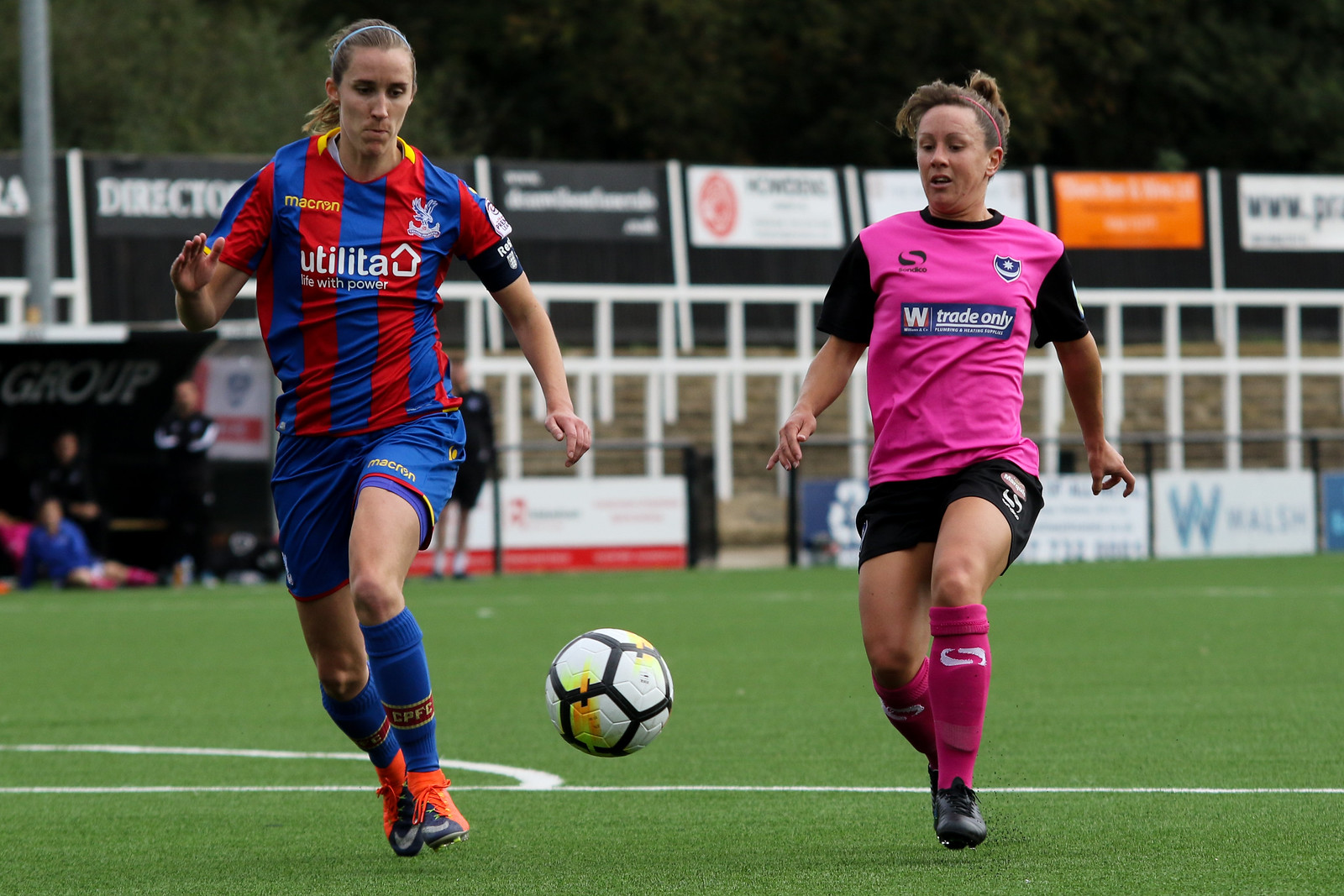The image captures two women soccer players in action on a green soccer field. The player on the right is wearing a pink top with black sleeves, accented by a horizontal blue bar on the front that says "W, trade only" in white text. She pairs this with black shorts, pink socks adorned with a white design, and black soccer shoes. Her hair is tied up in a ponytail, secured with a thin headband. The player on the left sports a blue and red vertically striped shirt that reads "Utilita" with a small house symbol underneath. She complements her outfit with blue shorts, blue socks featuring a red stripe, and orange and black shoes. Her hair is styled similarly, tied up and kept in place with a headband. Between them is a black-and-white soccer ball with yellow accents, bouncing slightly above their calf height as they both run after it. The background includes a green field with white painted lines, some empty bleachers, advertisements, and a few blurry figures: three people sitting near the back wall—one on the ground and one standing, while another sits on a bench. The scene is clearly set outdoors.